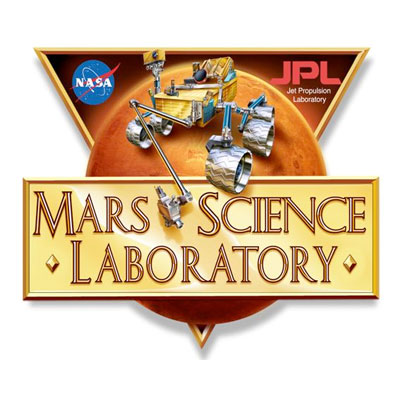In this detailed illustrative graphic, the focal point is an upside-down triangle with a vivid gold three-dimensional frame. Positioned within the triangle is a striking depiction of the planet Mars, predominantly colored reddish-brown. Centered on Mars is a meticulously drawn or photoshopped Mars rover, featuring metallic wheels, a gold-hued body, and various appendages including a camera and robotic arms. 

The top left corner of the triangle showcases the iconic blue NASA logo with a red swoosh and white lettering. Meanwhile, in the top right corner, the initials "JPL" appear in red, and directly beneath, the text "Jet Propulsion Laboratory" is presented in white. A rectangular gold bar, with the inscription "Mars Science Laboratory" carved into it, overlaps the Martian image. Additional details include two small gold diamond shapes flanking the text "Laboratory" in the gold bar. The overall setting of the image seems to emphasize the collaborative efforts of NASA's Jet Propulsion Laboratory in exploring Mars with the Mars Science Laboratory rover.